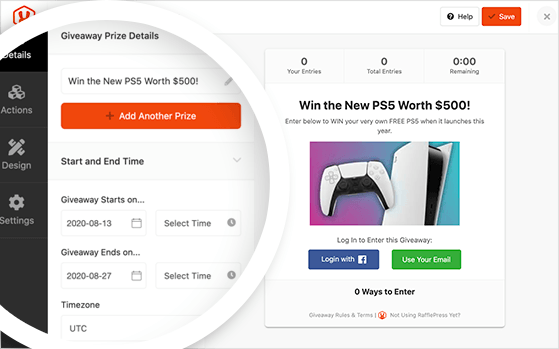This is a screenshot from a website detailing a giveaway prize. The header announces "Giveaway Prize Details," prominently featuring a chance to "Win the New PS5 worth $500." Below this, a plus button allows users to "Add Another Prize." The giveaway details list a start date of 2020-08-13 and an end date of 2020-08-27, with the time zone specified as UTC. 

On the left sidebar, navigation links are labeled "Actions," "Design," and "Settings." To the right, various statuses are displayed, including "Your Entries," "Total Entries," and "Time Remaining," all showing zeros. The main section repeats the prize information: "Win the New PS5 worth $500. Enter below to win your very own free PS5 when it launches this year." 

An image within the screenshot includes an Xbox controller and a hand controller. Beneath the image, instructions prompt users to "Log in to enter this giveaway," with login options for Facebook or email. Currently, it shows "Zero ways to enter."